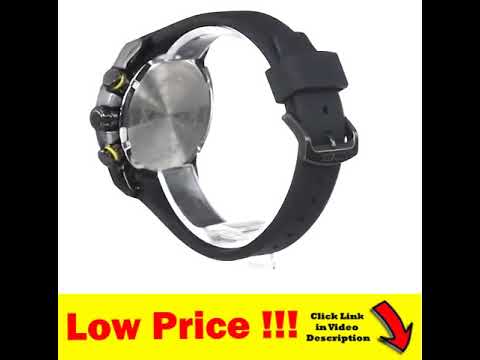This image is an advertisement for a wristwatch, focused on showcasing the back side and band of the timepiece. The photograph depicts the watch against a pure white background with vertical black bars framing the left and right sides. The watch has a closed, black rubber wristband featuring a stylized buckle and a circular plastic piece inside to maintain its shape. The back of the timepiece is silver, and three cylindrical knobs are located on the left side; the top and bottom knobs are a golden color, while the middle one is darker and slightly larger. The advertisement prominently displays a bright yellow rectangle at the bottom, flanked by the black bars, with red text that reads "Low price!!!" and "Click link in video description." This text is accompanied by a red arrow pointing downward, curving slightly to the right, emphasizing the call to action.